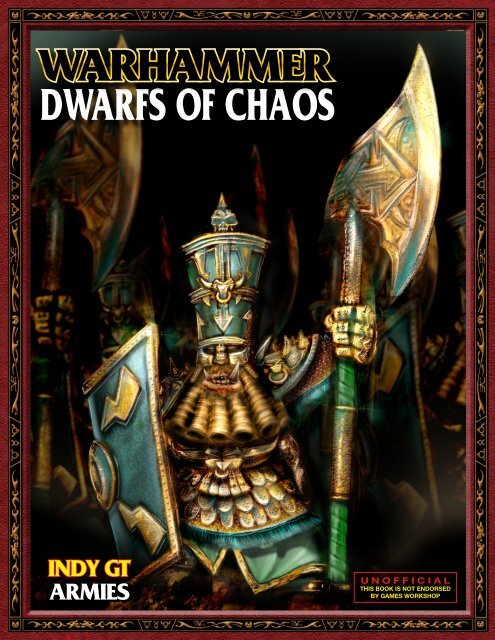This image is a detailed book cover for "Warhammer: Dwarfs of Chaos." The style is computer-generated artwork featuring a central, highly detailed dwarf warrior. The dwarf, positioned front and center, is clad in elaborate blue and gold armor and wears a tall, cylindrical helmet adorned with a monstrous design and two front-facing horns. His long beard is intricately curled into five thick ringlets. He holds a green-and-bronze-banded halberd with a gold-colored blade in his right hand and a square, green and gold shield in his left hand. The dwarf also has armored gloves and shoulder spikes.

The cover has a red border with a black strip containing unique gold shapes and abstract designs. At the top left, the text "Warhammer" is outlined in gold, with "Dwarfs of Chaos" in bold white lettering. In the bottom left, "Indie GT Armies" is printed, with “Indie GT” in yellow and “Armies” in white. The bottom right corner features a disclaimer in red and yellow: "Unofficial. This book is not endorsed by Games Workshop." The background of the cover is predominantly black, with more dwarves similarly armored and weaponized, blending into the shadows.